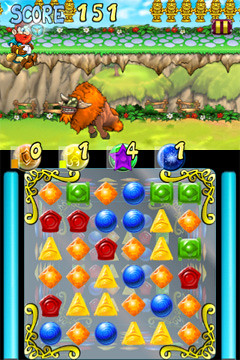This rectangular image captures a dynamic scene from a bejeweled puzzle game reminiscent of Bejeweled. The upper portion of the image features a buffalo adorned with a metal helmet, charging leftward across a lush grassy landscape. A cliff forms the backdrop, with a small red figure perched on the ledge's edge, adding an element of intrigue. In the top left corner, the word "Score" is displayed in blue text, and further towards the center, a yellow number "151" indicates the current score.

On the right side, six small gold figures suggest the remaining lives available in the game. The lower portion of the image centers around a large, vibrant puzzle grid filled with colorful jewels, where players must align matching shapes to create explosive combinations. At the top of this puzzle grid, four distinctive jewels are depicted: an orange jewel marked with a yellow zero, a yellow jewel with a yellow one, a purple star-shaped jewel featuring a yellow four, and a blue circular jewel also with a yellow one. These details create an immersive and detailed snapshot of the gaming experience.